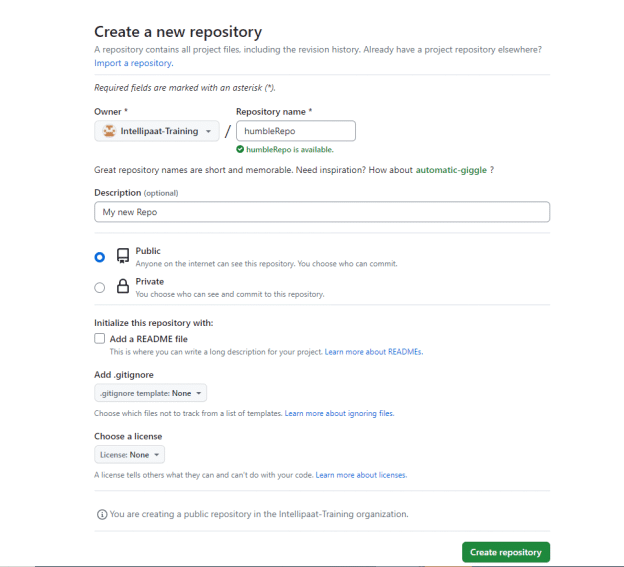#### Caption for Repository Creation Page:

The image depicts a webpage interface for creating a new repository. At the top, bold black letters announce "Creating a new repository." Below this heading, a subtext explains that "A repository contains all project files, including the revision history." 

For users who already have a project repository elsewhere, there's a blue hyperlink labeled "Import a repository." 

A gray line separates this section from the subsequent instructions. The next section informs that required fields are marked with an asterisk (*). The first field is labeled "Owner*" with a dropdown box, wherein "Intellipass Training" is selected. A forward slash follows the selection.

Adjacent to this dropdown box is a text box labeled "Repository name," with "humble-repo" entered. A green checkmark beneath the text box confirms that "humble-repo is available." Below the checkmark, a suggestion reads, "Great repository names are short and memorable. Need inspiration? How about 'automatic-giggle'?" The suggested name "automatic-giggle" is in green.

The next field, labeled "Description (optional)," contains an editable text bar with the placeholder "My new repo."

Two selectable boxes follow. The first is labeled "Public" with a note that "Anyone on the internet can see this repository. You can choose who can comment, commit." The second box is labeled "Private," indicating "You can choose who can see and commit to this repository." In this instance, the "Public" option is selected.